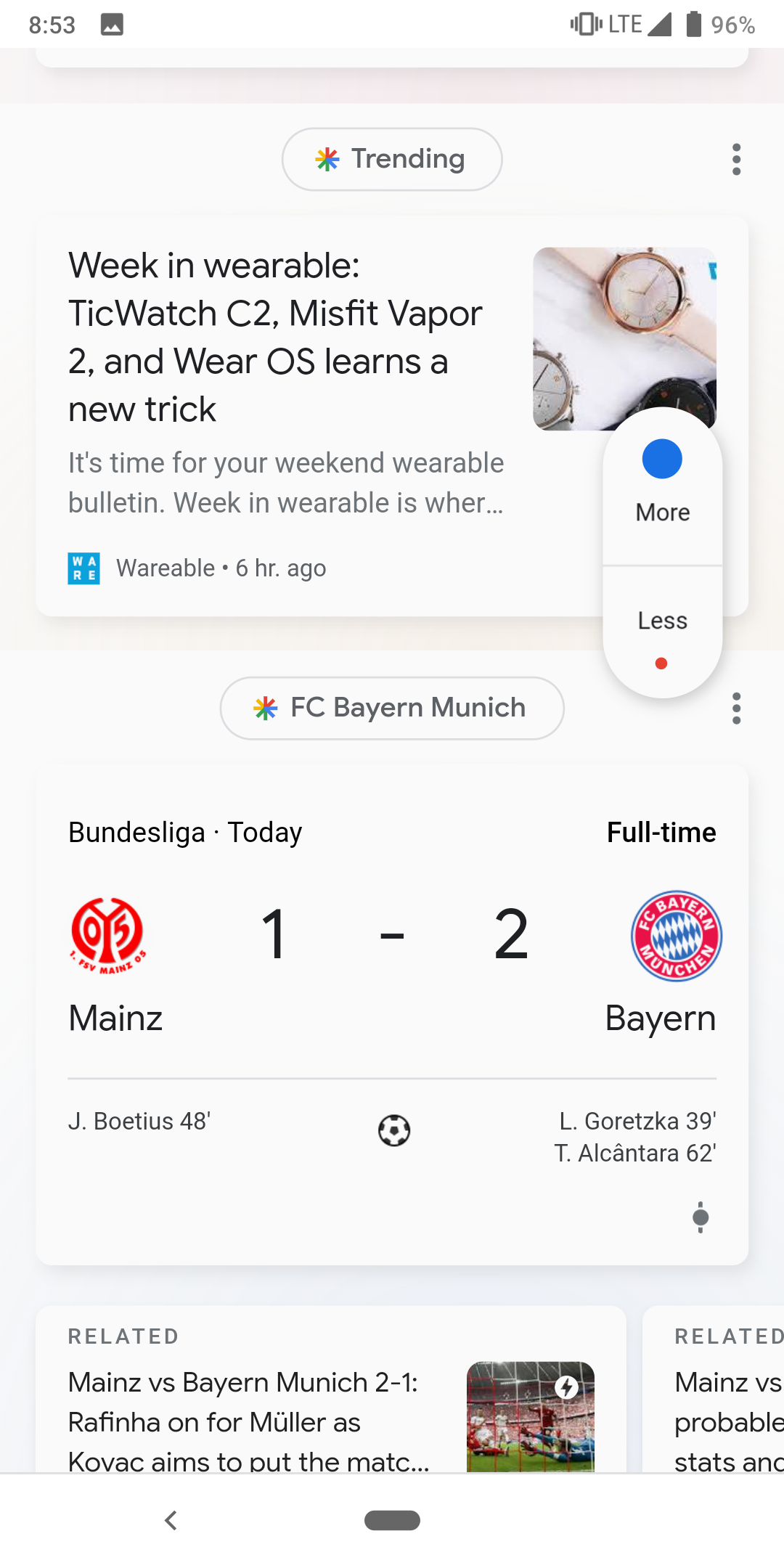In the screenshot from the Ether app on a smartphone, the "Trending" section is prominently displayed at the top, marked by a button labeled "Trending" with a Google star icon to its left. The star features the recognizable Google colors: red, blue, green, and yellow.

Below this, there is an article titled "Weekend Wearable Bulletin," with the subheading "TicWatch C2, Misfit Vapor 2, and Wear OS learns a new trick!" The article is categorized under "Wearable" and was posted six hours ago. Adjacent to the article, there are images of three smartwatches: a gold one, a black one, and a silver one. Additionally, there is an expandable section controlled by buttons labeled "More" (blue circle) and "Less" (red circle).

The second item in the trending list features the same Google star and pertains to an FC Bayern Munich match result. It displays the score "Mainz 1 – Bayern 2" with match details: Mainz's goal by J. Poitras at 48 seconds, and Bayern's goals by L. Goretzka at 39 minutes and T. Alcantara at 62 minutes. Below, it mentions "Related: Mainz vs Bayern Munich 2-1" with Rafinha's commentary on Formula 1 as Kovac aims to push the match. Iconography for both teams is included; Mainz’s icon is red, and Bayern’s icon incorporates red, white, and blue colors.